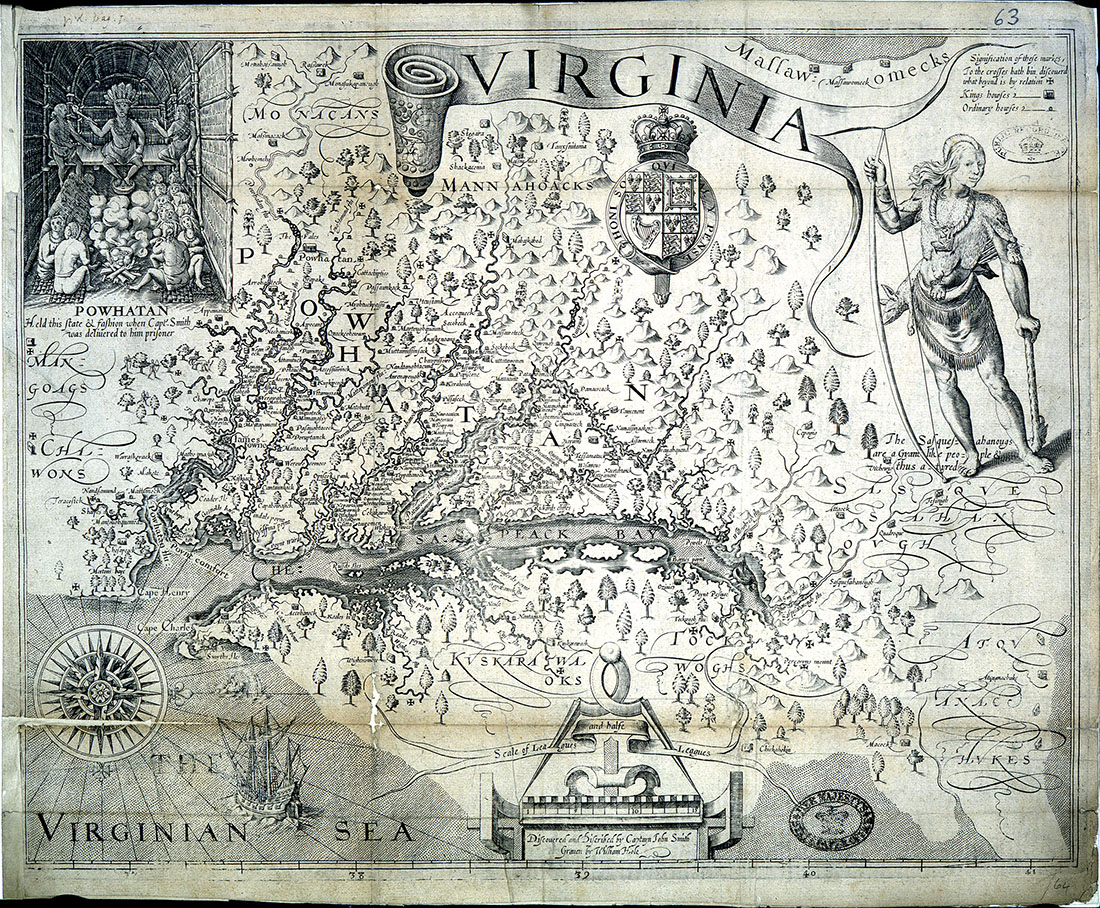This image features an aged, hand-drawn map of Virginia, likely dating back to the colonial era, well before the founding of the United States. The map, printed in black and white, showcases highly detailed line drawings and is in English. The map has been heavily aged, exhibiting yellowed paper and darkened creases from being folded, with tattered and worn edges barely visible within the photo frame.

Central to the map is a depiction of the Virginia Sea, labeled in the lower left corner. Accompanying this label is a detailed drawing of a large sailing vessel and a compass. The sea is surrounded by bays, rivers, trees, and hills, all meticulously illustrated. At the top of the map, a banner labeled "Virginia" stretches across, with a crest situated beneath it, though the crest’s details are somewhat unclear.

In the upper left corner, there is a portrayal of Powhatan Indians, suggesting a scene of worship in front of a statue. Meanwhile, the top right corner features an indigenous figure holding a bow in one hand and leaning on an axe or a staff, looking to the right. Additionally, there is some sort of structure, possibly a wall or building, depicted at the bottom center of the map. The intricate elements and historical value of this map make it a significant representation of early Virginia.